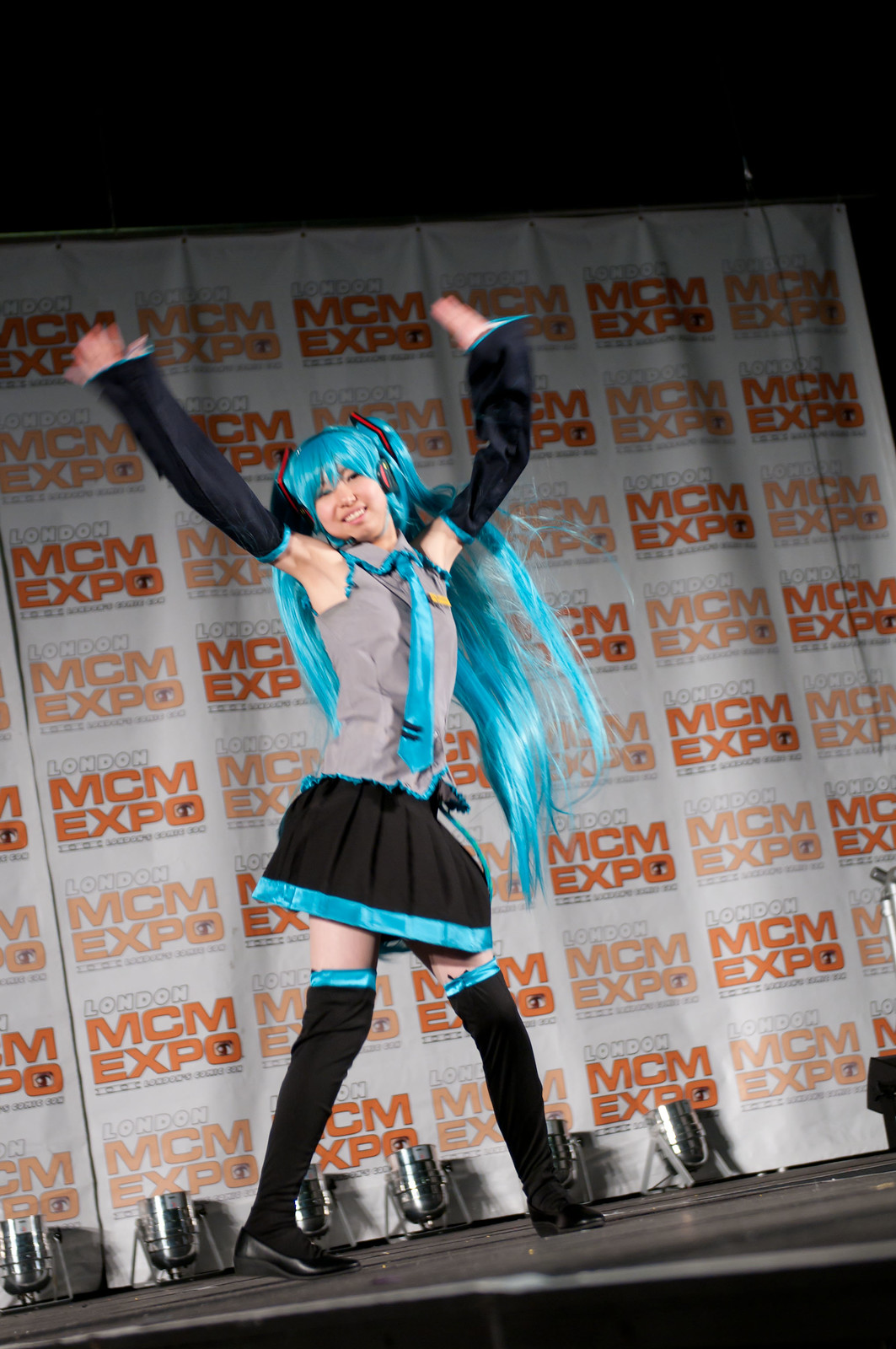The photograph captures a vibrant scene of a young woman, possibly a pop star or cosplayer, performing energetically on stage at the MCM Expo. Her long, blue hair with bangs complements her joyful expression as she dances with both arms raised high. Her outfit includes a gray sleeveless tank top, a black skirt with a blue stripe at the bottom, and thigh-high black socks also featuring a blue stripe at the top. She accessorizes with arm sleeves and a headpiece equipped with a microphone. On her feet are black shoes. The stage is illuminated by several spotlights aimed upward, adding a dynamic flair to her performance. Behind her, a large banner repeats the "MCM Expo London" logo in alternating yellow and orange colors against a white background, setting a lively backdrop for the event. The overall scene is one of excitement and entertainment, capturing the essence of the MCM Expo.